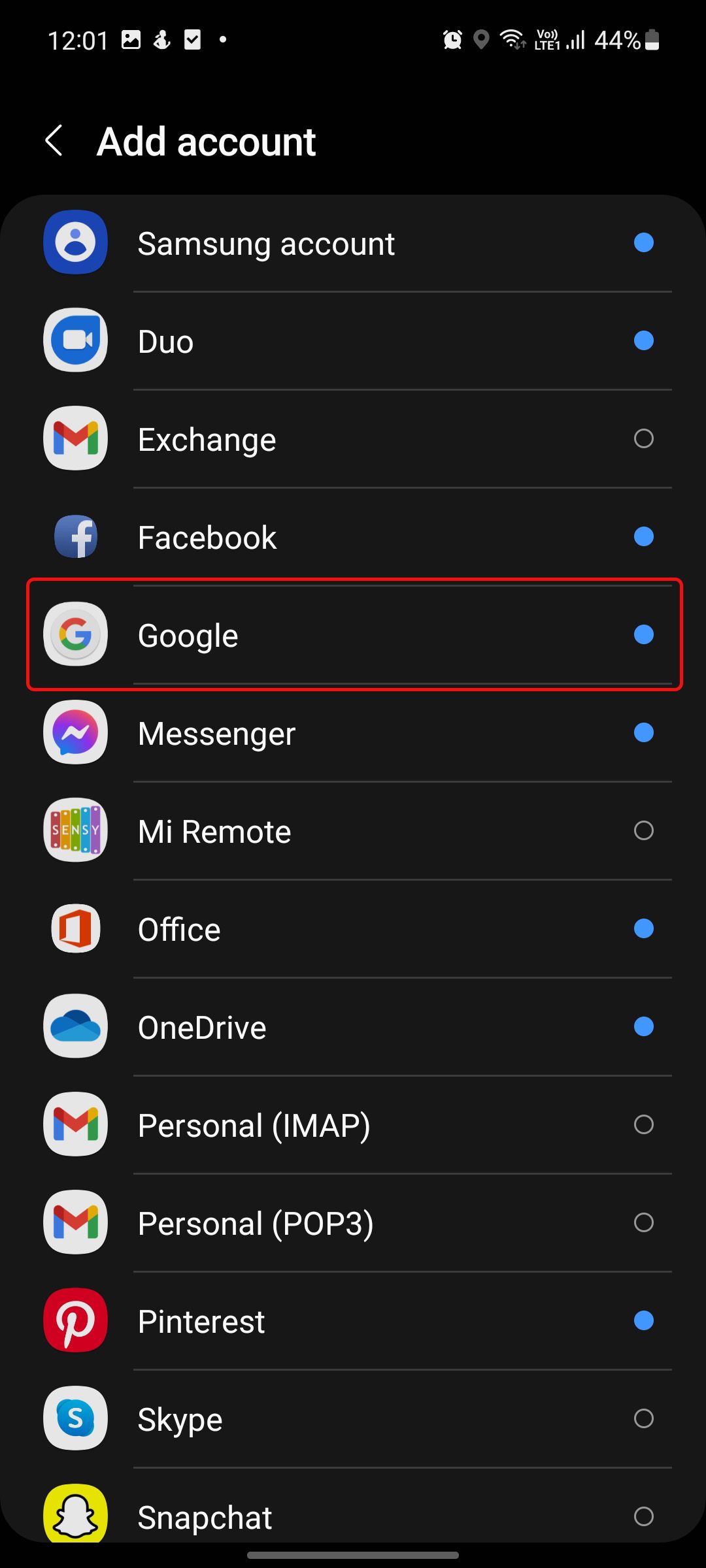This image is a detailed screenshot from a mobile device showcasing a settings menu. The background of the screenshot is black, and several status icons are visible at the top of the screen. On the left, there is a time display that reads "12:01," followed by various icons including a home button, a person running, a checkbox, and a dot. These are indicative of different app notifications. On the right side, an alarm clock icon is present, indicating an alarm is set. Below that, there are indicators showing that the location services are turned off, Wi-Fi is connected with full signal strength, and the device is connected to a network labeled "B-O(LTE1)" with full cellular bars. The battery level is displayed as 44%.

At the very top of the screen, a header reads "Add account" with a back button on the left. Below the header is a list of accounts that can be added to the phone. The accounts listed are: 

1. Samsung account (selected)
2. Duo (selected)
3. Exchange (not selected)
4. Facebook (selected)
5. Google (selected, highlighted with a red box)
6. Messenger (selected)
7. MI Remote (not selected)
8. Office (selected)
9. OneDrive (selected)
10. Personal IMAP (not selected)
11. Personal POP3 (not selected)
12. Pinterest (selected)
13. Skype (not selected)
14. Snapchat (not selected)

Next to the chosen accounts, blue filled circles are visible on the right, while unselected accounts are indicated with empty circles.